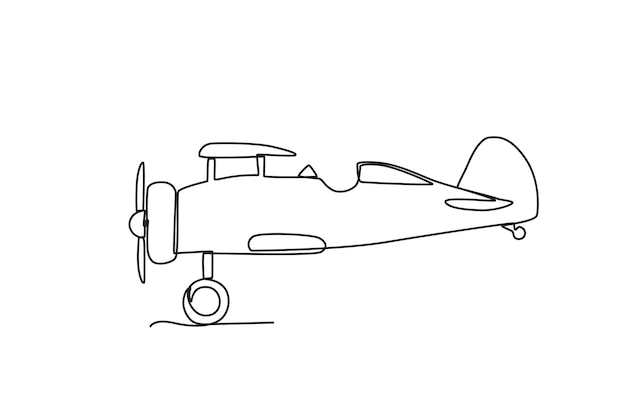This is a black-and-white pencil drawing of a small, single-engine airplane on a white background. The illustration is simple and cartoonish, emphasizing clear, clean lines. The airplane is depicted in a side view, facing to the left. It features a front propeller and a singular wheel positioned beneath the fuselage. There's a small triangular window atop the cockpit area, and an indentation suggesting a seat. The plane has a top wing extending backward, with a tail wing at the rear. The wheel is drawn as a circle connected by a line to the plane, with another line beneath it implying the ground. Despite the minimalistic approach, the drawing captures the essence of a personal, one-person aircraft.